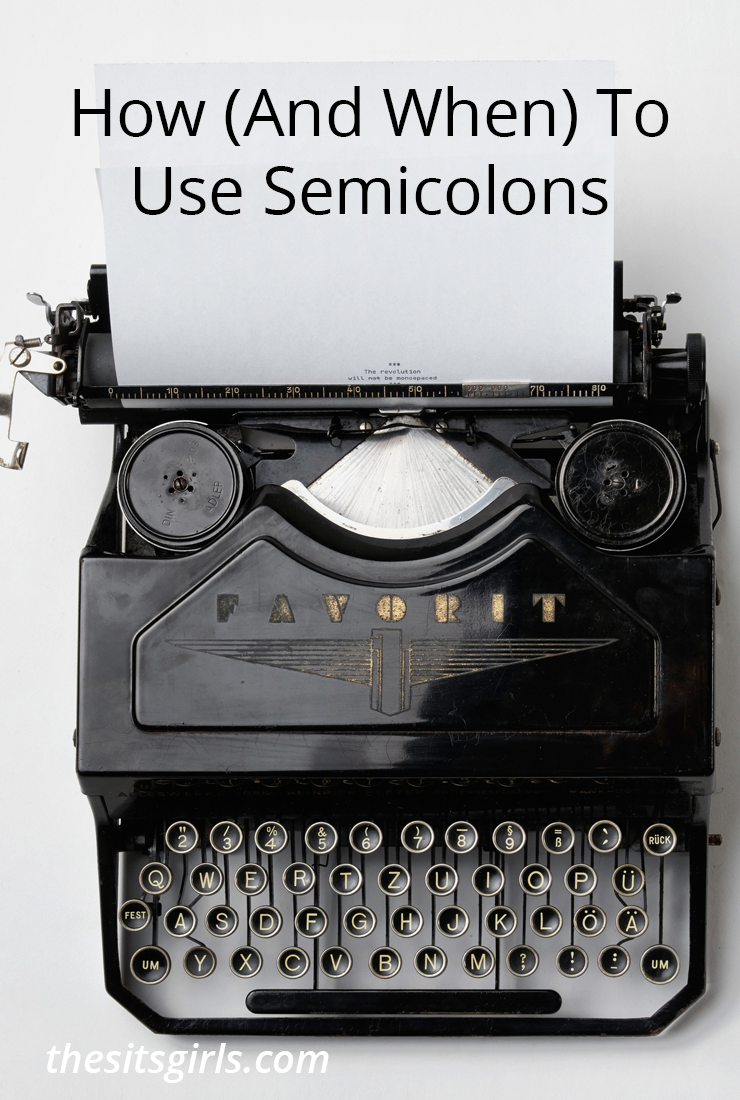The photograph showcases a top-down view of an antique black typewriter placed on a light gray flat surface. The typewriter, distinguished by its slightly unconventional design, is labeled with the brand "FAVORIT" in gold text that is fading. Below the brand name is a logo that resembles a wheel with golden wings. The typewriter features multiple round keys with gold lettering for letters and numbers. These keys appear to float above a hollow section, with visible space bars reinforcing its vintage aesthetic. Mounted on the typewriter are two ink drums positioned beneath a piece of white paper. Overlaying the paper is the text "how (and when) to use semicolons" in black print. In the bottom left corner of the image, a watermark reads "TheSitGirls.com."